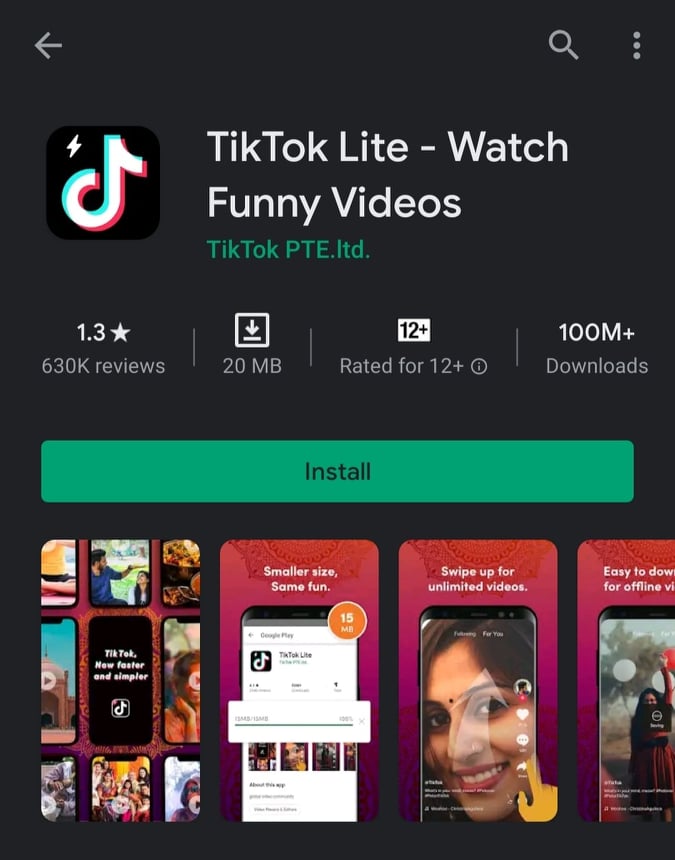Screenshot from a Mobile Device Showing the Google Play Store Describing TikTok Lite

In this cropped screenshot from a mobile device, the Google Play Store application is open, highlighted by a distinctive black background. At the top, a grey back arrow, a search magnifying glass, and three vertical dots are clearly visible. The focal point of the screenshot is the app "TikTok Lite," with its tagline, "Watch funny videos." On the left, the app's logo resembles a backwards musical note with a small white lightning icon.

The app's statistics are prominently displayed: it has garnered 630,000 reviews with an average rating of 1.3 stars. The download size of the app is 20 megabytes, and it is rated suitable for users aged 12 and above. To date, the app has been downloaded over 100 million times. 

A large green "Install" button stands out, inviting users to download the app. Below the install button, four screenshots from within the TikTok Lite application are showcased, advertising its diverse functionalities and features.